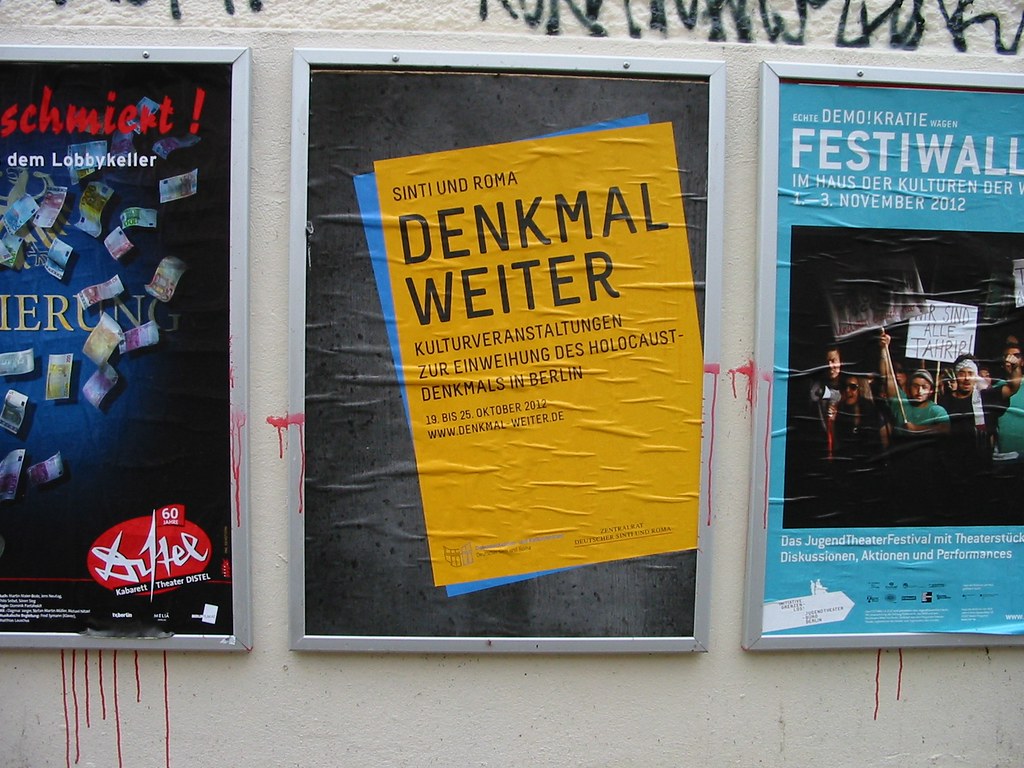The photograph captures a series of three posters affixed to a white concrete wall, partially covered with blue-gray graffiti. The posters seem to be German advertisements, with a distinctive focus suggesting historical and social contexts.

The central poster is prominently featured, entirely visible without any cutoffs. It has a black background with striking yellow and blue elements. The bold text "Denkmalwetter" — indicative of a German origin — is visible, and beneath it, words related to the Holocaust, possibly mentioning "Sinti" and "Roma," are present. This poster's detailed colors include shades of pink, yellow, and blue.

On the right, another poster stands out with a robin's egg blue background featuring an image of protesters holding white banners. This poster, labeled with "Festiwahl," includes a date, "November 3rd, 2012," and is predominantly blue and white.

The leftmost poster is the least visible, partially cut off by the edge of the photo. It transitions from a black to royal blue background with gold text and depicts flying money. There's evidence of red splatters, likely paint, streaked across this poster and dripping down, creating a stark visual effect.

Overall, the photograph portrays a mix of cultural, socio-political, and commercial themes, reflecting a vibrant yet gritty urban landscape.